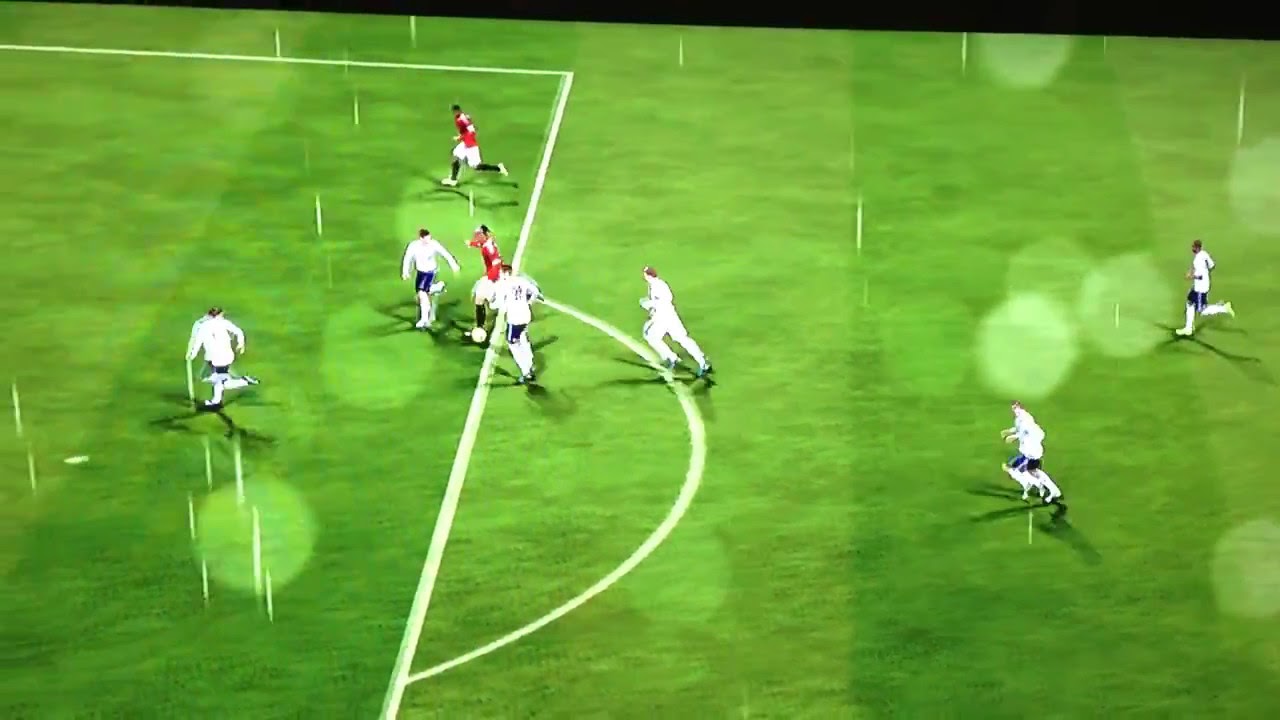The image shows an overhead view of a soccer match on a horizontal-rectangular field, with grass in various shades of green that suggest it might be artificial turf. The field has distinct white lines, including the goal area boundary and a circle outside of it, and a black border, possibly indicating a surrounding track. The scene includes spotlights illuminating the field. The image appears somewhat blurry and has a cartoonish or video game-like quality, potentially due to glare, rain, or reflections from a glass partition, suggesting it might have been taken from a viewing area indoors.

On the field, there are six players in white uniforms defending their goal, and two players in red uniforms. One red-uniformed player at the top of the image seems to be positioning for a shot at goal, closely trailed by two white-uniformed players. Another red-uniformed player appears to have the ball and is surrounded by three white-uniformed opponents attempting to intercept it. The overall scene conveys an intense moment in the soccer match with a distinct digital or reflective visual characteristic.